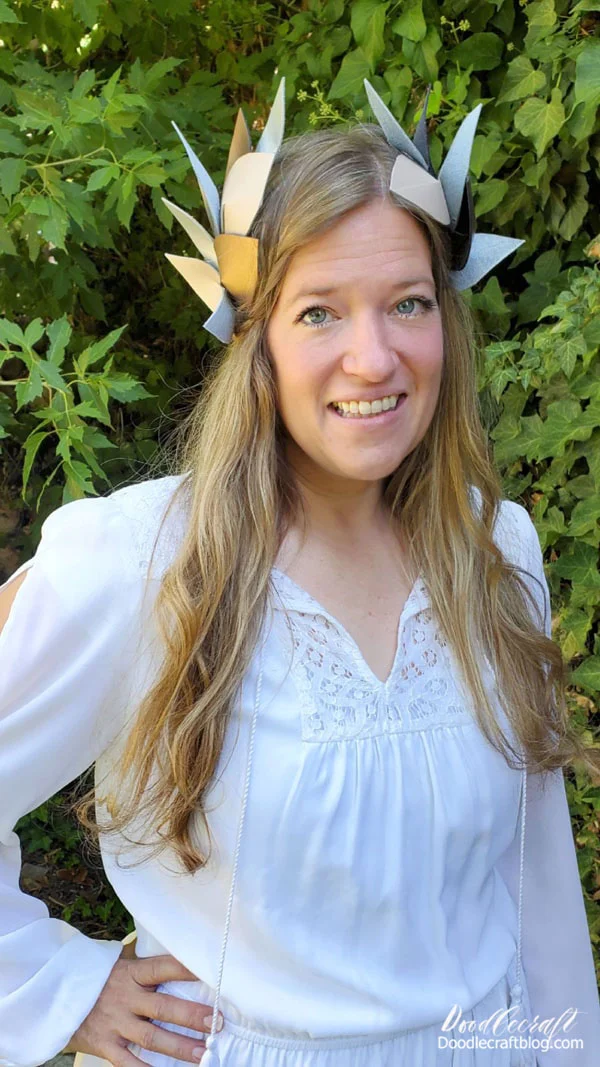The photograph captures a Caucasian model with long, wavy blonde hair cascading past her chest, smiling softly for the camera. Her striking bluish-green eyes are framed by fanned-out lashes, and she wears a flowing white dress adorned with intricate embroidery along a V-neckline and on the sleeves, which feature cutouts that reveal her skin. Her left hand rests confidently on her hip while her right arm hangs gently by her side. Adorning her head, two spiked crowns made of brown and olive cardboard pieces create a regal, wreath-like effect. She stands before a lush backdrop of vibrant greenery, likely a large bush or tree, with hints of brown dirt visible beneath the foliage. The image, set in daylight, carries a watermark in the lower right corner that reads "Doodlecraft" in cursive, above the URL "doodlecraftblog.com".